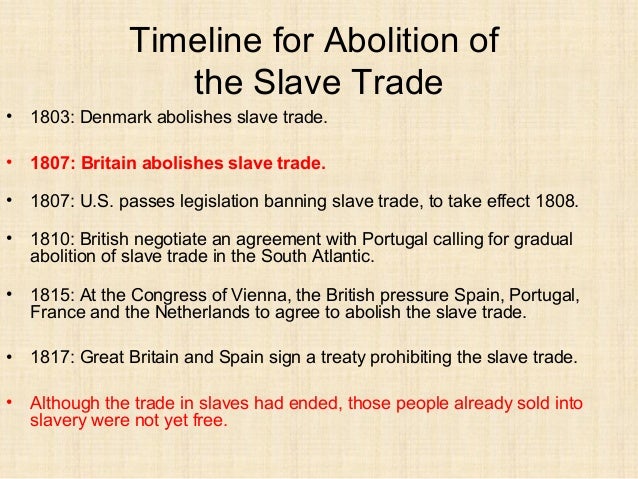The image features a detailed timeline on the abolition of the slave trade, presented as text over a pinkish tan, faded background, resembling an old document or perhaps a PowerPoint slide. The title, "Timeline for Abolition of the Slave Trade," is prominently displayed at the top in bold. The content lists significant dates and events: In 1803, Denmark abolished the slave trade; in 1807, Britain did the same; that same year, the U.S. passed legislation to end the slave trade effective in 1808. By 1810, the British had negotiated with Portugal for the gradual abolition of the trade in the South Atlantic. In 1815, at the Congress of Vienna, Britain pressured Spain, Portugal, France, and the Netherlands into agreeing to abolish the slave trade. Lastly, in 1817, Great Britain and Spain signed a treaty prohibiting the trade. Despite these milestones, the text notes the somber reality that those already enslaved were not yet free. The layout of the text is meticulously spaced and easy to read, featuring a color palette of tan, black, white, and red.